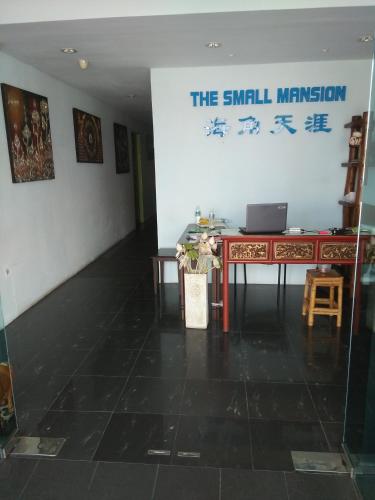The image depicts a small, dimly lit room that appears to be the entrance to an office or an exhibit. The room features a black tile floor and white walls, with high hat lights on the ceiling that are off. On the far wall, blue text reads "The Small Mansion" with some Asian characters underneath. There is a brown, intricately patterned, Asian-style desk with an open gray laptop on it. Adjacent to this, forming an L shape, is another desk containing water bottles, papers, and a large vase with flowers. A stool and a chair are positioned at the desk. To the left is a darkened hallway leading to more rooms, adorned with various pieces of artwork. The room is viewed through clear glass pane doors, adding to its exhibit-like ambiance.